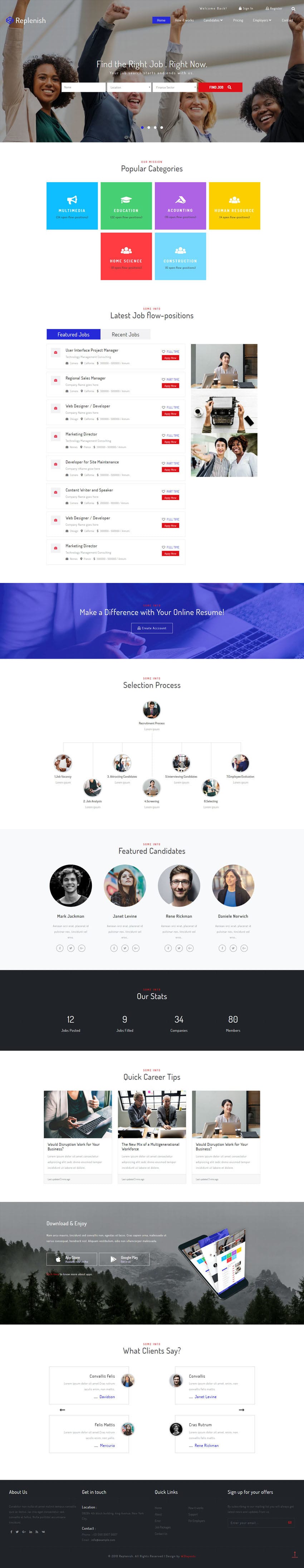The screenshot captures a long and narrow segment of someone's computer screen, featuring a variety of visual elements arranged vertically. At the very top of the screen, there's an image depicting four people - three females and one male - standing with their arms raised in front of a brown-colored building. Below this image, three horizontal white bars are visible; they appear to be entry fields, possibly for typing information, accompanied by a conspicuous red "Search" button.

Directly beneath these bars is a white section containing six colored boxes arranged in two rows. The first row consists of four boxes colored blue, green, purple, and yellow. The second row has two boxes, one red and the other blue. Following this section, text appears in a column, though it is blurred and difficult to decipher. Next to this column of text are multiple red buttons aligned vertically.

A purple border runs horizontally across the middle of the screen, separating the upper sections from the lower content. Below this boundary, there are several small, circular images, each accompanied by text underneath. Additionally, several small circle icons with accompanying text are visible.

Further down, there's a black rectangular section with three square images underneath it. The background transitions to an image of mountains that spans the width of the screen, with some text positioned underneath. The very bottom of the screenshot features a dark black rectangle, completing the layout.